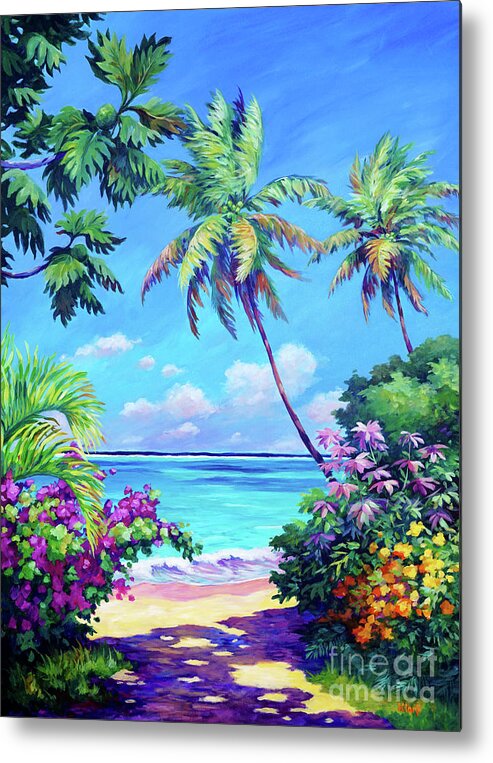This art piece, possibly a print on canvas or a watercolor painting, vividly captures a serene beach setting reminiscent of Florida or Hawaii. The scene depicts a walking path of brown sand leading directly to the water, flanked by lush tropical plants. On either side of the path, there are two slender palm trees – one situated in the center and the other on the right. The foreground is adorned with vibrant shrubbery, featuring beautiful purple, lavender, yellow, and orange flowers intermingled with wispy leaves. The crystal-clear water stretches far out, displaying a stunning gradient of bluish-green shades, which transition into darker blue hues toward the horizon. The sky overhead is a beautiful mix of light blue and deep blue, dotted with a few white, puffy clouds. This painting’s detailed and realistic art style, complete with subtle shadows of the trees on the ground, invites viewers on an immersive journey down the sandy path to the tranquil beach. Marked with "Fine Art America" in the bottom right, this piece is an exquisite representation of a tropical paradise.